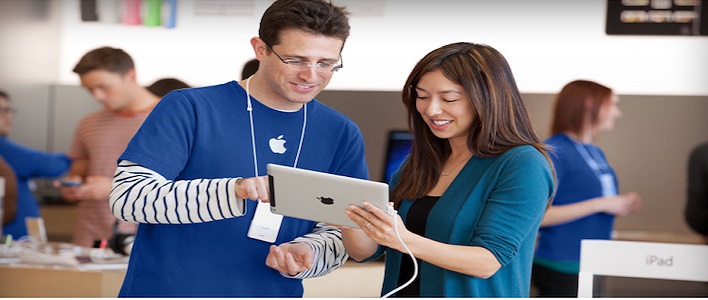In this lively scene captured at an Apple Store, a friendly employee, distinguished by his blue Apple t-shirt emblazoned with the company's insignia and a blue and white striped shirt peeking out at the neckline, assists a customer. The employee, a bespectacled Caucasian man with spiky brown hair, sports a lanyard likely bearing his ID. He attentively engages with a Latina woman, who is immersed in the iPad she is holding, which remains connected via its charger. Her broad smile reflects her excitement, complemented by her long dark hair, turquoise cardigan, and black tank top.

In the dynamic backdrop of the busy store, other patrons can be seen interacting with a range of devices. To the left, a Caucasian man with brown hair and a reddish striped shirt closely examines another device on a nearby table. Further behind them, another Apple employee, identifiable by her blue t-shirt and lanyard, stands slightly blurred. This woman, with reddish hair, gazes off towards the right of the image, contributing to the bustling yet orderly atmosphere of the store. This photograph vividly illustrates a typical moment of customer interaction and engagement within the welcoming environment of an Apple Store.